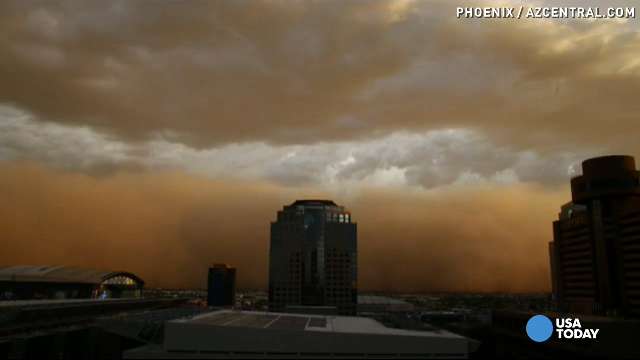This photograph, likely a magazine cover or page, prominently features a high-rise building set against a dramatic, orangey sky, suggesting it's either sunset or early evening. The sky above is filled with large white and gray clouds, partially obscuring the sun and casting a backlit glow. The scene is somewhat dark, making it difficult to discern the exact features of the buildings. In the center stands a large skyscraper, with additional high-rises and various shorter buildings scattered throughout the background, primarily to the left and right. The top right of the image is marked with the text "phoenix-arizonacentral.com" and "azcentral.com," while the bottom right corner features the USA Today logo accompanied by a small blue circle.